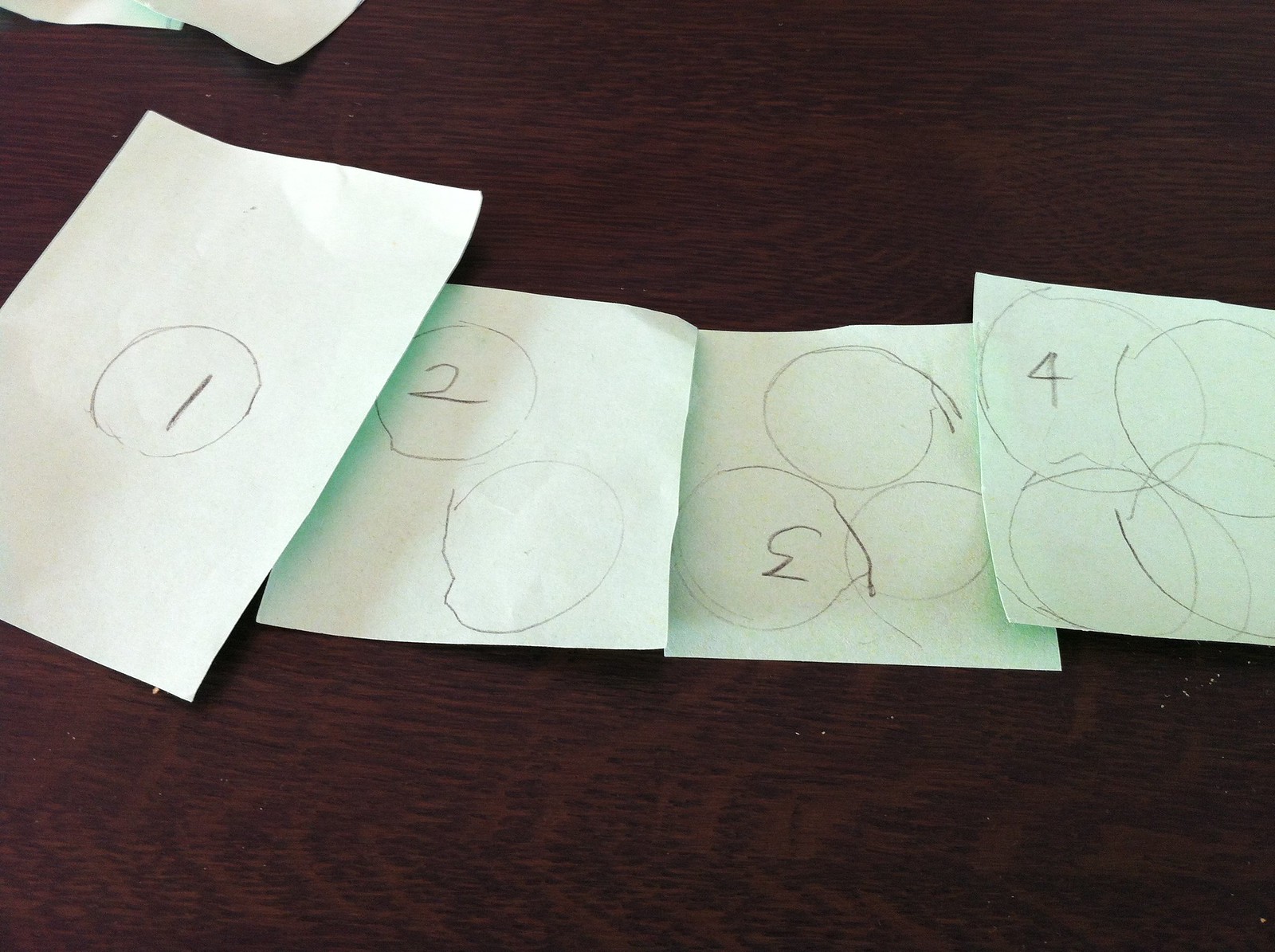On a wooden surface lie four pieces of paper, each a shade of green, seemingly created by a child. The first sheet features a single pencil-drawn circle with the number "1" inscribed in the center. The second sheet displays two circles and the numeral "2." The third sheet has three circles, though the maker appeared to struggle with some of them, each accompanied by the number "3." The fourth and final paper stands out with its four intersecting circles and the number "4." All the artwork is done in pencil, showcasing the child's developing skills.